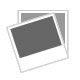The image showcases a small, square-shaped glass bottle with a gold cap, containing a red or amber-brown liquid, likely perfume or cologne. The bottle features elegant etchings on its sides. Positioned to the lower left, the bottle is complemented by a sophisticated round container set above it, crafted from polished stone with a white base featuring brown or red veining. This container includes a separate lid with a silver metal handle. Inside the container is a precise insert, possibly foam or plastic, designed to snugly fit and hold the perfume bottle. The background of the image is a light gray, providing a neutral backdrop that accentuates the luxurious appearance of the items.